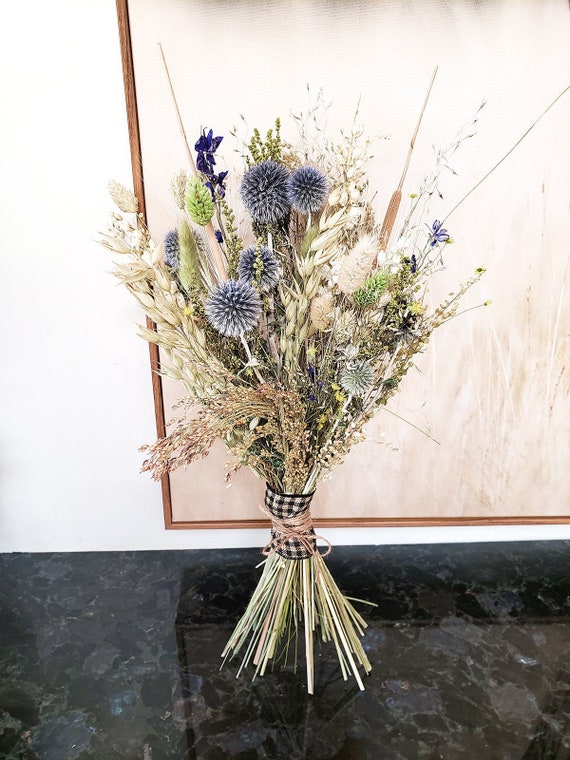The image depicts a tall, intricately tied bundle of dried wildflowers placed on a shiny black granite countertop. The bouquet, devoid of any vase, is secured with a black and white checkered cloth and string. It features a diverse assortment of flowers, including blue and purple blossoms, straw-like stems, green foliage, wheat-like elements, and cattail-like protrusions, all cohesively arranged. Behind the bouquet, there's a white wall adorned with a framed painting that adds a subtle, neutral background. The painting is characterized by a tan hue with white brushstrokes, and the wooden frame highlights it elegantly. The overall scene is accentuated by the reflection of the bouquet and part of the painting on the glossy countertop, enriching the setting with an airy yet earthy ambiance.